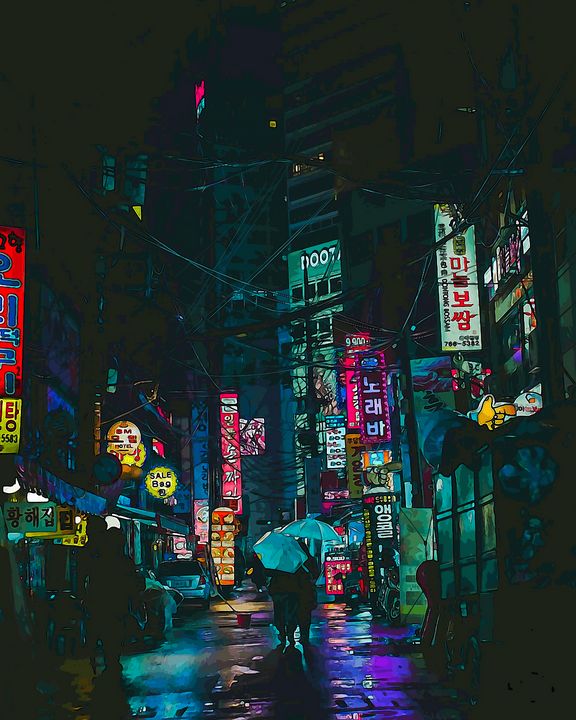This painting captures a vibrant, nocturnal cityscape, likely set in an Asian metropolitan area such as Tokyo or Seoul, characterized by its narrow, wet street reflecting the glow of neon lights from numerous storefronts and signs. The street is vividly brought to life with a spectrum of neon colors—hot pink, white, red, yellow, purple, and green—illuminating signs adorned with Asian characters, possibly Korean or Japanese. These storefronts are lined tightly on both sides of the street, with market awnings adding to the dense, bustling atmosphere. Overhead, telephone wires crisscross the top third of the scene, enhancing the urban feel.

In the foreground, two silhouetted figures walk away from the viewer, holding aqua or white umbrellas that contrast sharply with the dark, wet surroundings. The street, slick and shiny from recent rain, mirrors the vibrant neon, creating a dynamic, almost shimmering effect across the pavement. In the far background, a towering skyscraper looms, its presence felt through faintly lit windows and deep shadows.

The art style appears to utilize watercolor, lending the scene a fluid, dreamlike quality, with the predominance of black making the neon signs and wet reflections all the more striking. This detailed composition not only highlights the everyday human activity in a bustling night market but also showcases the interplay of light and shadow in a modern urban landscape.